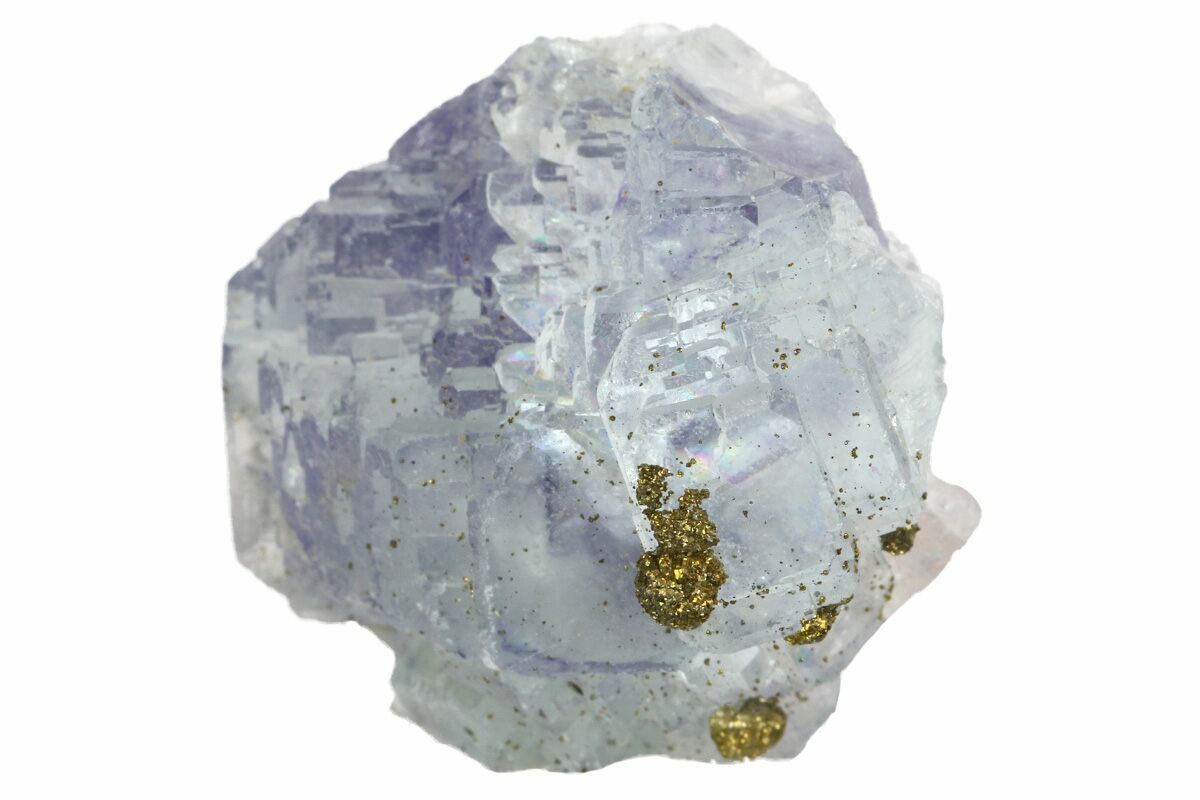This image showcases a captivating piece of quartz, notable for its transparent quality and inherent beauty. The quartz, though small and unpolished with a rough exterior, features several intriguing characteristics. Scattered across its surface are three distinct clumps of lustrous gold, which add a unique and striking contrast to the clear mineral. Additionally, the quartz displays speckles of gold on one face, further enhancing its visual appeal. This unrefined gem, with its natural inclusions and imperfections, exemplifies the raw elegance of nature's mineral formations.